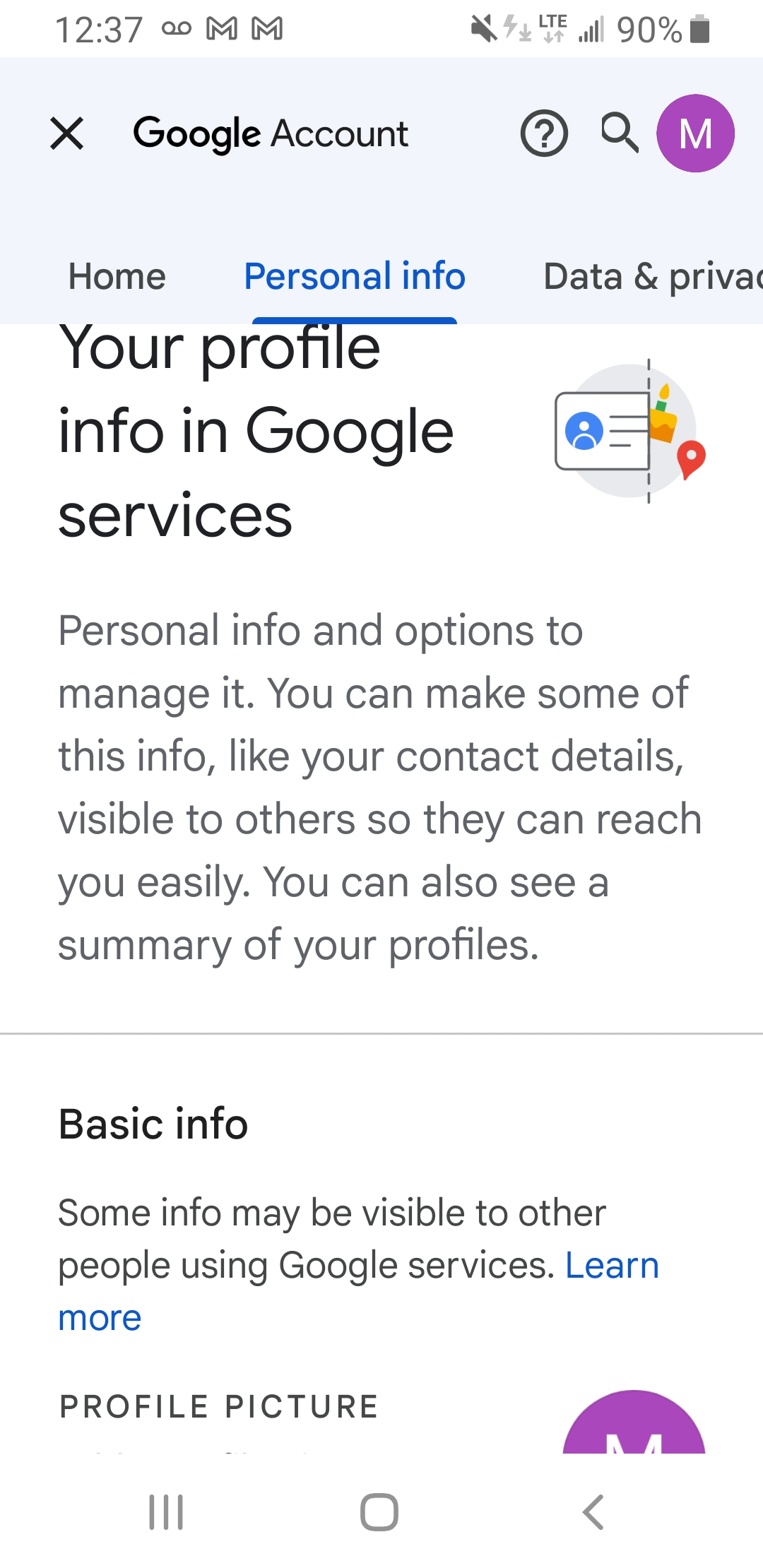Screenshot of a smartphone displaying a Google Services information page. At the top of the screen, the status bar shows the time (12:37), a voicemail symbol, two email icons, a muted ringer symbol, LTE connectivity, and a 90% battery level. The main section begins with the header "Google Account" accompanied by an "X" on the right and the letter "M" inside a purple dot. Below that, the navigation bar includes options labeled "Home," "Personal Information," "Data & Privacy," with "Personal Information" highlighted in blue. 

The highlighted section reads "Your profile info in Google services" next to an infographic. The text below describes options for managing personal info, contact details, and profile visibility, emphasizing the ability to make some information visible to others for easy contact. A line separates this section from the bolded "Basic info" heading, which informs users that some information may be visible to others using Google services. A blue "Learn more" hyperlink is provided. At the bottom, a partially visible profile picture is accompanied by a cut-off letter "M" and a navigation menu icon with three bars and an arrow on the left.